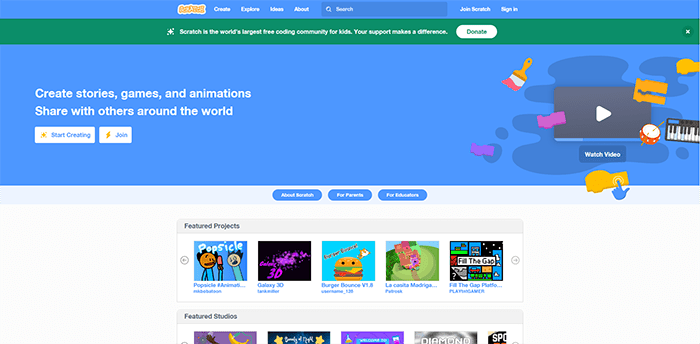On a vivid blue background at 200% zoom, the image features a centered display with "Scratch" outlined in yellow and white at the top. Beneath it, navigation options are listed: "Create," "Explore," "Ideas," "About," a search bar, "Join Scratch," and "Sign in." A description follows, highlighting that Scratch is the world's largest free coding community for kids, and emphasizes the importance of user support with the message "Your support makes a difference." A "Donate" button is also present.

The image encourages users to "Create stories, games, and animations, share with others around the world, and start creating or join." To the right, a "Watch Video" button is available. There are various items scattered, including different shapes that are not clearly identifiable but suggest objects like a watch, a keyboard, a drum, and a paintbrush. Additionally, a monitor is displayed to watch the video.

Below this section, featured projects and featured studios are showcased, with several cartoon-style characters designed to appeal to kids prominently displayed.